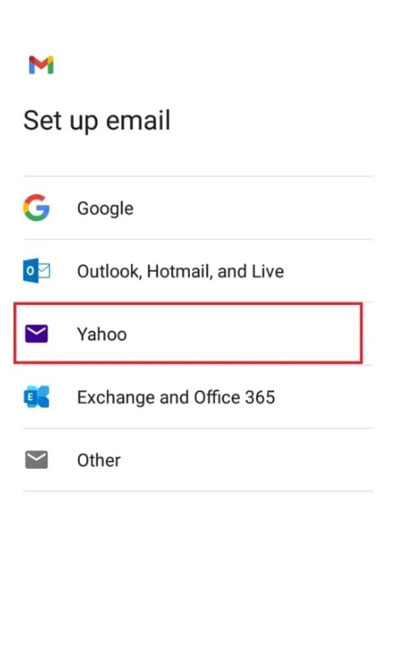The image is a screenshot from a website featuring a white background. At the top, there is a stylized letter "M" with its left leg in blue, the central part in red, the upper part in orange, transitioning to yellow at the tip, and descending to green. Below the "M," the text "Set Up Email" is displayed in black font with a capital "S." Further down, there is a line followed by a Google logo comprising a rainbow-colored "G" next to the word "Google" in capitalized font. Underneath, the words "Outlook, Hotmail, and Line" are listed, succeeded by "Yahoo" which is accompanied by a purple envelope icon with a red border. The options "Exchange" and "Office 365" are also listed, along with a gray envelope icon labeled "Other." The first letter of each major word is capitalized, and the rest of the image remains predominantly white.